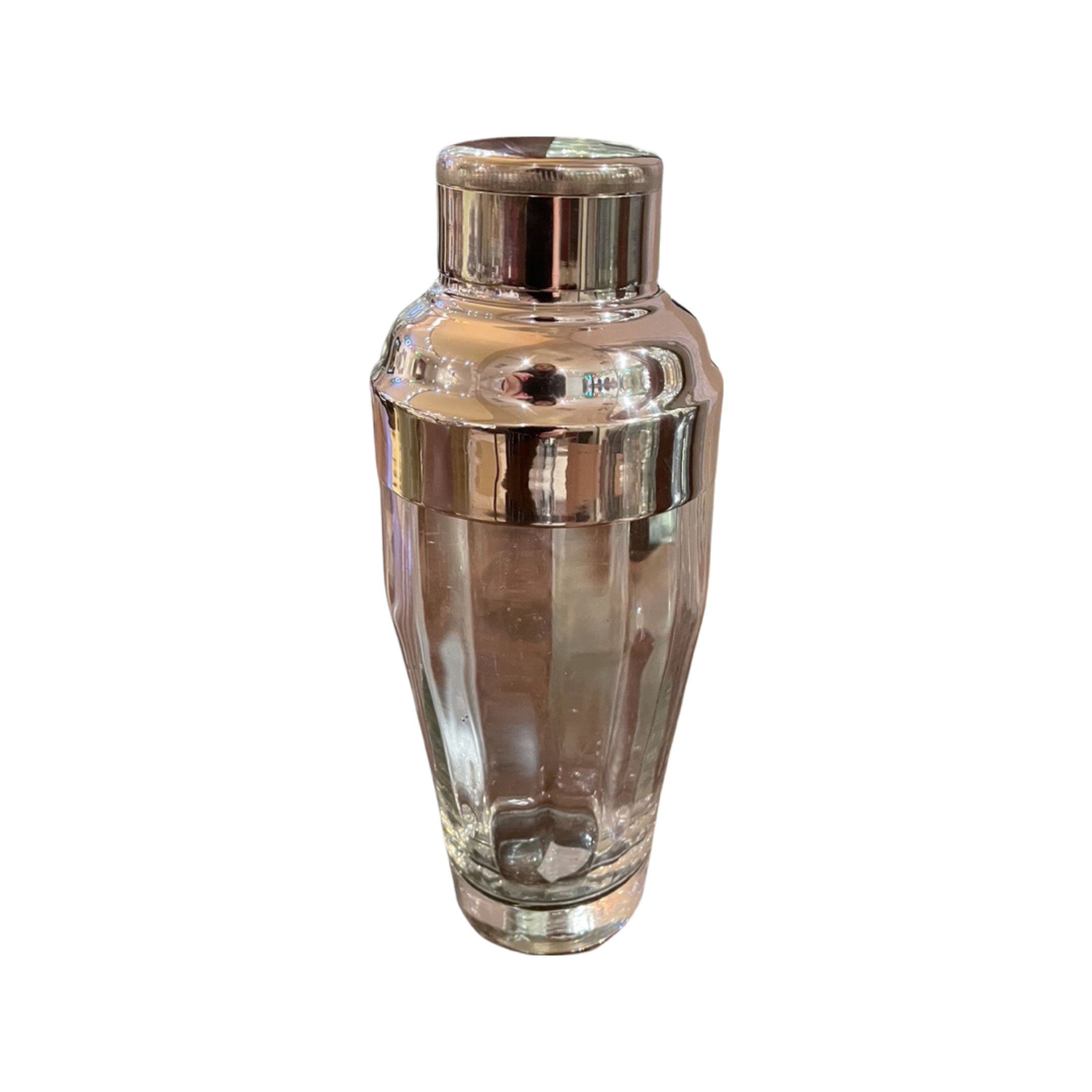This detailed photograph showcases a shiny, brown glass bottle resembling a vase or an urn. The bottle is predominantly narrow at the base and wider towards the top, culminating in a round, cap-fitted lid adorned with metallic-like elements. These elements are shiny, adding a reflective sparkle to the overall appearance. Additionally, there are vertically running marks on the cap. The bottle's translucent quality is emphasized by its reflective surface, capturing parts of the surrounding environment. A distinctive gold strip encircles the middle section, enhancing its decorative appeal. The bottle appears empty, allowing clearer visibility through the bottom section, suggesting a combination of glass and metal materials. The entire setup stands out against a pristine white background.